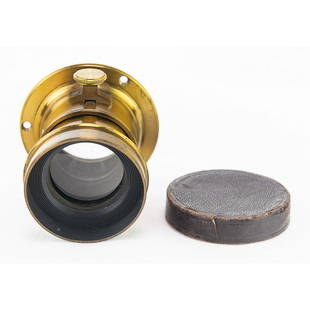In this image, a brass or bronze eyepiece, possibly from an antique camera or telescope, is laid on a tabletop. The eyepiece is a hollow, circular metallic structure with a clear, slightly curved lens at its center, encased in a smaller metal cylinder that appears to have a rubber coating inside. It features two rivet holes for mounting and a tiny turnable knob on the top, indicating some integral adjustment mechanism. Adjacent to the eyepiece, on its right, rests a round lens cap, crafted from textured brown leather, and designed to fit over the eyepiece, presumably for protection. This cap is slightly bumpy, features a small button, and indentations around its outer edge.